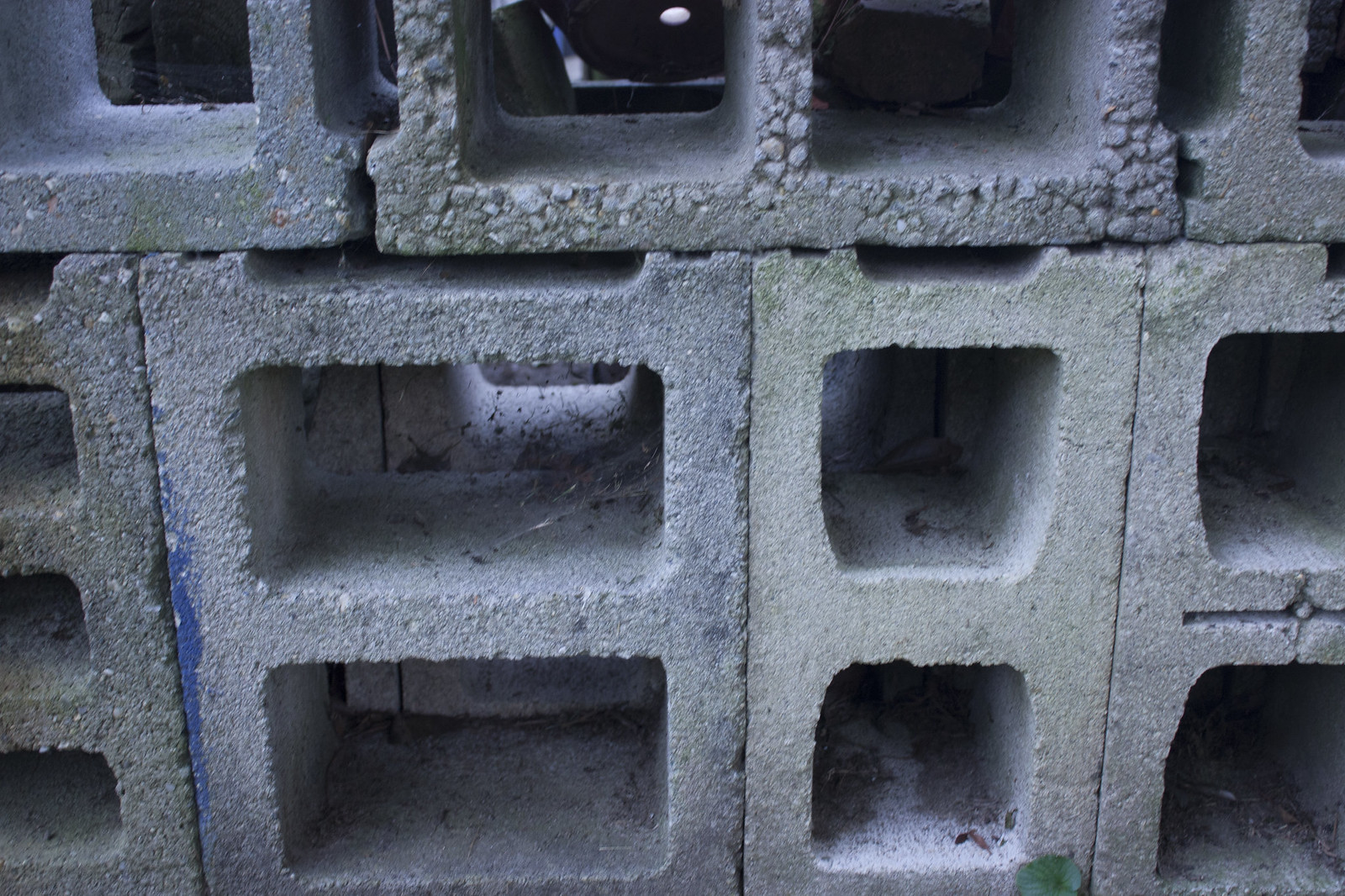The image depicts a weathered and dusty stack of cinder blocks. At the bottom of the picture, there are four vertically positioned cinder blocks, gray in color with each having two holes in the center. These blocks appear to be worn, with traces of paint and spider webs indicating age. Stacked on top of these are three more cinder blocks laid horizontally, side by side. While most of the cinder blocks are similar in size, there is one notably wider block in the bottom row, second from the left, which also has two holes. In contrast, the block on the far left has three openings instead of two. The scene is set outdoors in daylight, and the blocks, varying slightly in shades of gray, appear to be composed of smaller rocks and pebbles combined into larger stones, reminiscent of materials used before constructing a building.